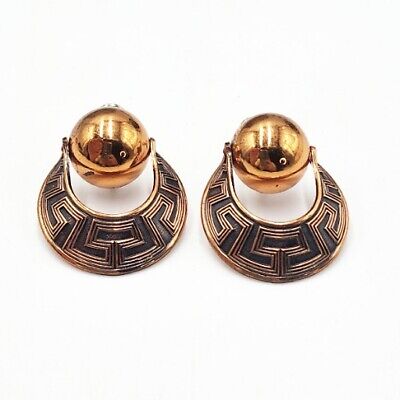The image features a close-up of two intricate gold and black objects, set against a plain white background, suggesting they might be for sale. Each object consists of a gold base adorned with geometric designs. Rising from the base is a black platform with textured gold lines that resemble a maze, adding depth and complexity to the design. At the top of each platform sits a reflective gold ball, shaped almost like a horseshoe, capturing the reflection of the photographer taking the picture with their phone. The primary colors present are gold, black, and white, providing a striking contrast and highlighting the intricate details and craftsmanship of the objects, which appear to be either decorative items or possibly earrings.